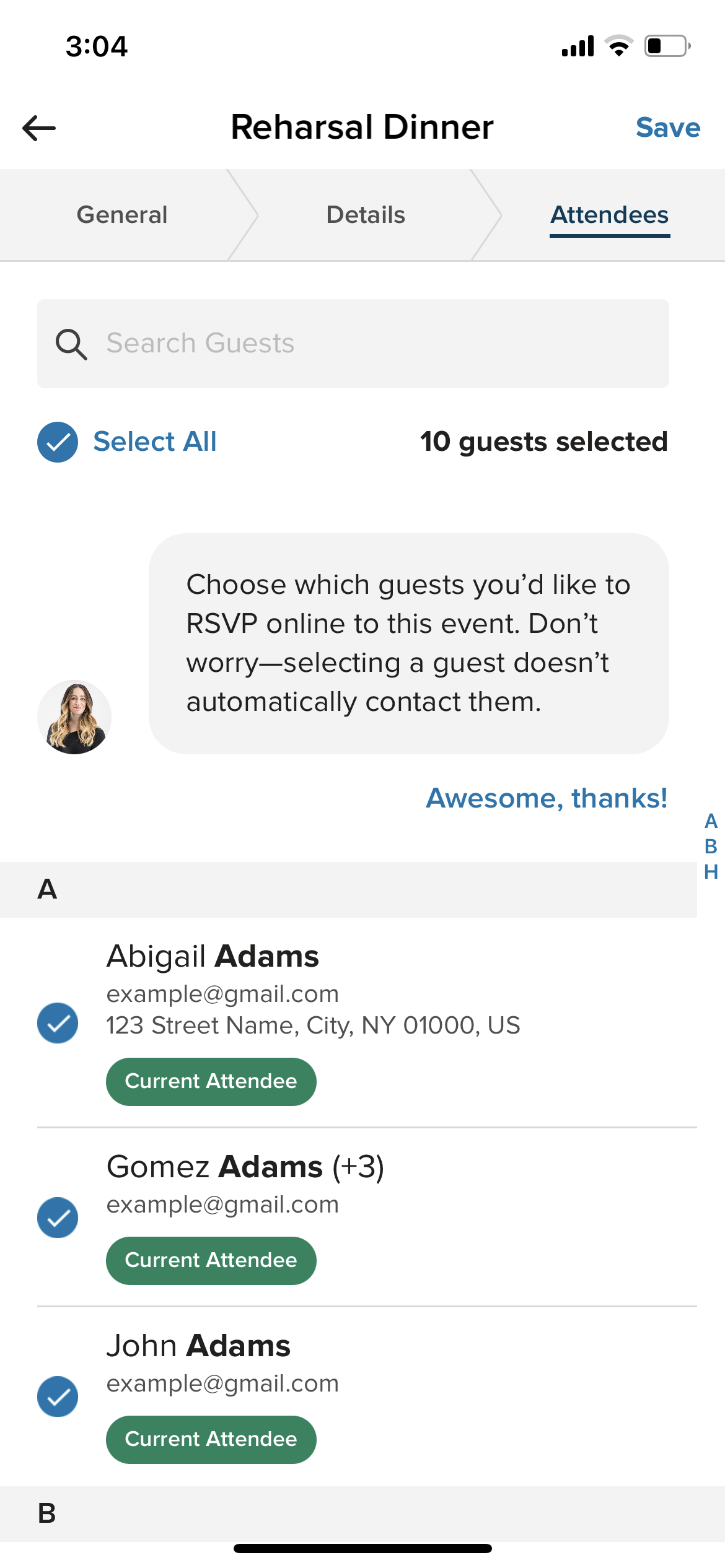The image depicts a phone screen displaying the interface of an event management application, specifically for a rehearsal dinner. The top section of the screen shows the heading "Rehearsal Dinner" with navigation tabs below, labeled "General," "Details," and "Attendees." The "Attendees" tab is currently selected.

Beneath the navigation tabs, there is a search bar labeled "Search Guest," displayed in gray. Below the search bar are options "Select All," indicating 10 guests have been selected. The note, "Choose which guest you'd like to RSVP online to this event. Don't worry, selecting a guest doesn't automatically contact them," is displayed with an accompanying comment, "Awesome, thanks."

A profile picture of a woman with long, wavy brown and blonde hair, wearing a black shirt, is visible. The guest list is organized alphabetically, starting with the letters A, B, and H. Under the letter "A", three names are listed: Abigail Adams, Gomez Adams, and John Adams. Each entry shows an example email address (example@gmail.com) next to a blue check mark. Green buttons labeled "Current Attendee" are situated beneath each name.